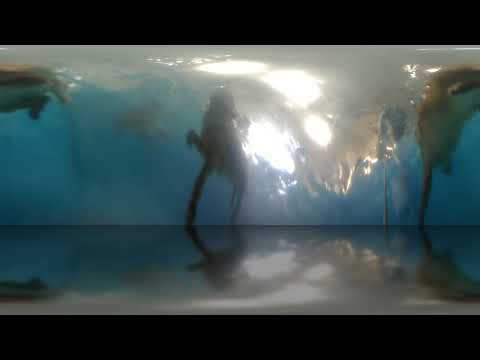The image appears to be a blurred and distorted photograph, likely taken with a fisheye lens or in panorama mode, of an underwater scene within an aquarium or fish tank. The water is primarily blue, and flat, bluish walls form the background, with a distinct line marking the boundary between the bottom and the wall. White lights are visible at the top, their reflections casting shadows and adding to the difficulty in discerning details. In the center of the tank, a creature resembling a frog stands upright with its long, slender legs extended. To the left, another similar creature, possibly a frog, hovers near the top of the frame with its legs close to its body. On the right, yet another creature, which may or may not be a frog, appears to have one leg up and one down, somewhat resembling a mouse. Additionally, there seems to be a dark, pixelated human hand entering the frame from the left. The scene is shadowy and grainy, making it challenging to identify the exact nature of the creatures within the tank.